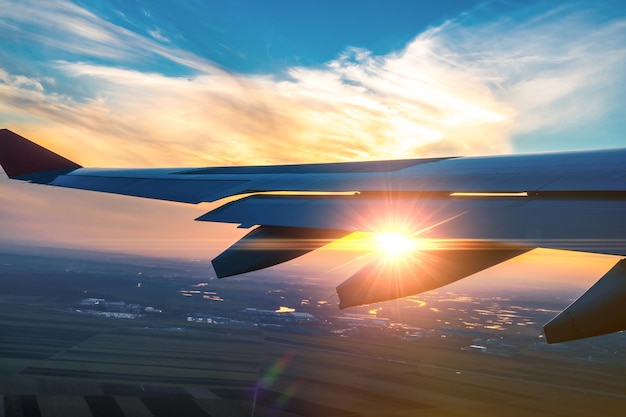The image captures a breathtaking scene of a plane taking off into the sunset. Dominating the foreground is the plane's left wing, ascending as the plane gains elevation. The setting sun, positioned towards the center right of the photograph, blazes through the wing, creating a striking solar flare effect. The sky above is a vibrant blue, adorned with large, white clouds tinged with hues of orange and red, signaling the twilight hour. Below, traces of a city with blurred lights appear hazy, alongside patches of empty land and grass. The contrast between the serene sky and the bustling ground below adds depth to this mesmerizing aerial view.